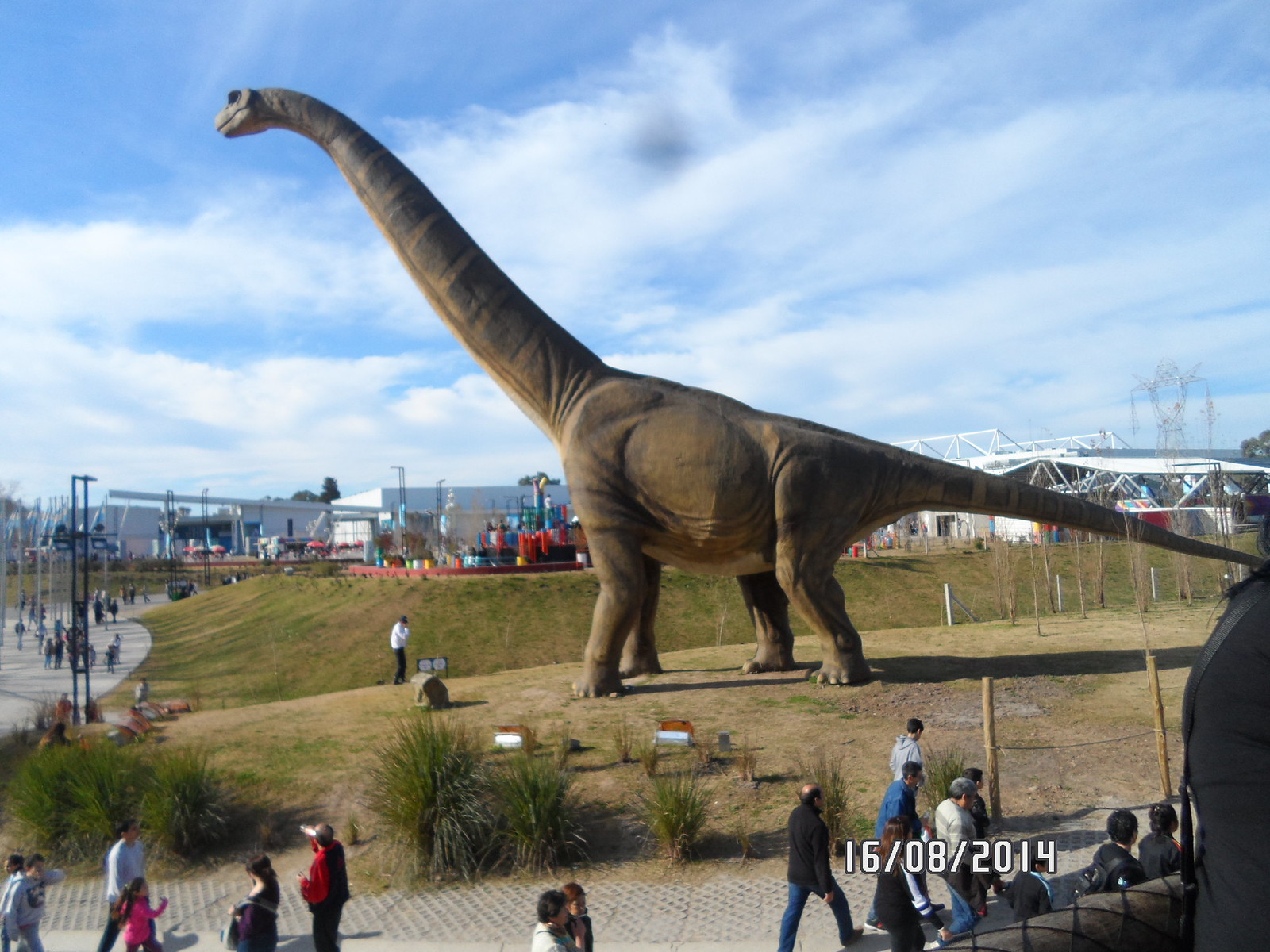In this vibrant and bustling park scene, dated 16/08/2014, a very large dinosaur statue with a really long neck and tail dominates the center, standing on its four sturdy legs. This olive green and brownish colored dinosaur attracts numerous visitors, who are wandering on grayish pathways around it. One man appears particularly interested in a sign near the dinosaur. The sky above is bright blue, adorned with puffy white clouds, adding to the lively atmosphere filled with people playing with their children. In the background, a playground and a big white building can be seen, further enriching this dynamic snapshot of a busy and engaging recreational space. Verdant green plants encircle the dinosaur, enhancing the natural feel of the park.